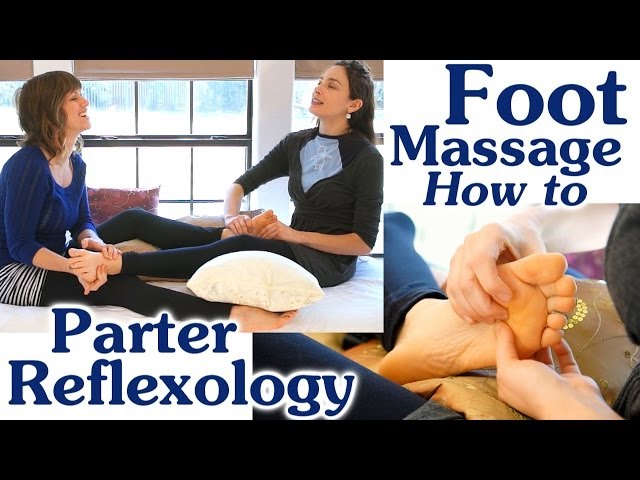The image is an instructional poster on foot massage techniques, featuring the title "Foot Massage: How To" in a dark blue serif font located at the upper right. On the bottom left, it also reads "Parter Reflexology" in the same font. The main photograph showcases two women seated on the floor, facing each other, and smiling while massaging each other's feet. One woman, who appears to be in her late 20s, is wearing a black shirt and dark blue pants with her dark hair adorned with a white earring. The other woman, seemingly in her late 40s, is dressed in a light blue sweater paired with a black and white striped skirt and leggings. A pillow rests on top of the younger woman's foot, adding to the relaxed atmosphere. In the background, a window with a pillow propped on the windowsill can be seen. On the bottom right of the image, there is a close-up shot showing the woman in the blue shirt's foot being massaged, with detailed emphasis on the curvature and tension as the other woman's hands press into it. The overall scene conveys a sense of enjoyment and relaxation shared between the two women.